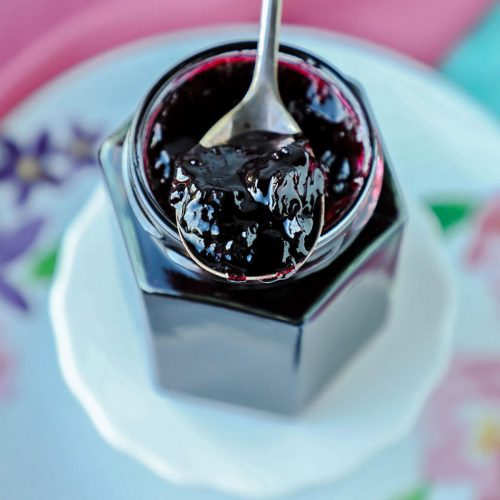The image depicts a detailed and aesthetically arranged scene from a top-down view. At the center, a hexagon-shaped glass jar filled with dark purplish-red jelly, likely grape or blackberry, sits without its lid. Emerging from the jar, a round silver teaspoon is scooping up a generous serving of the perfectly gelatinous jelly. The jar itself rests on a plain white, smaller round glass plate, which in turn is placed on a larger white dinner plate adorned with a floral pattern featuring purple and pink flowers with yellow centers and green leaves. The majority of the square image is occupied by these plates. The background is purposefully blurred, casting the focus solely on the intricate setup and the spoonful of jelly. A pink object, possibly a cloth, appears in the blurred background, adding a hint of color contrast in the top part of the image.